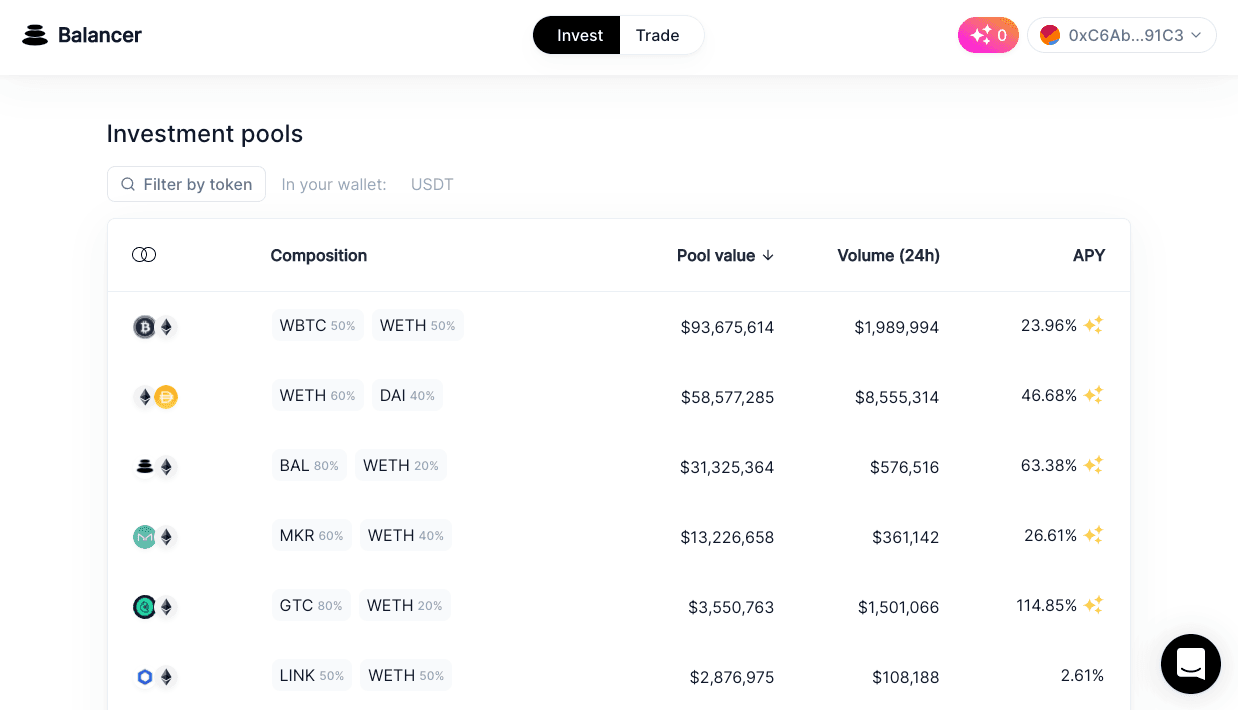Website screenshot of "Balance Balancer," a platform designed for investment and trading. On the left side of the image, the word "Balancer" is prominently displayed. The category "Invest" is highlighted in black, emphasizing its active selection over "Trade." To the right, a section labeled with the alphanumeric code "OX C6AB...91C3" features a small color-coded button in red, orange, and blue. Adjacent to this, a pink and orange circular icon is visible. 

This section lists various investment pools which users can filter by tokens in their wallet, including USDT. The table includes columns for Composition, Value (in USD), Volume (24H in parentheses), and APY (Annual Percentage Yield). 

The specific tokens available in this user's wallet include WBTC, WETH, BAL, MKR, GTC, and LINK. Each token entry shows its dollar value, trading volume in dollars, and APY in percentages, providing a detailed snapshot of the wallet's investment standing.